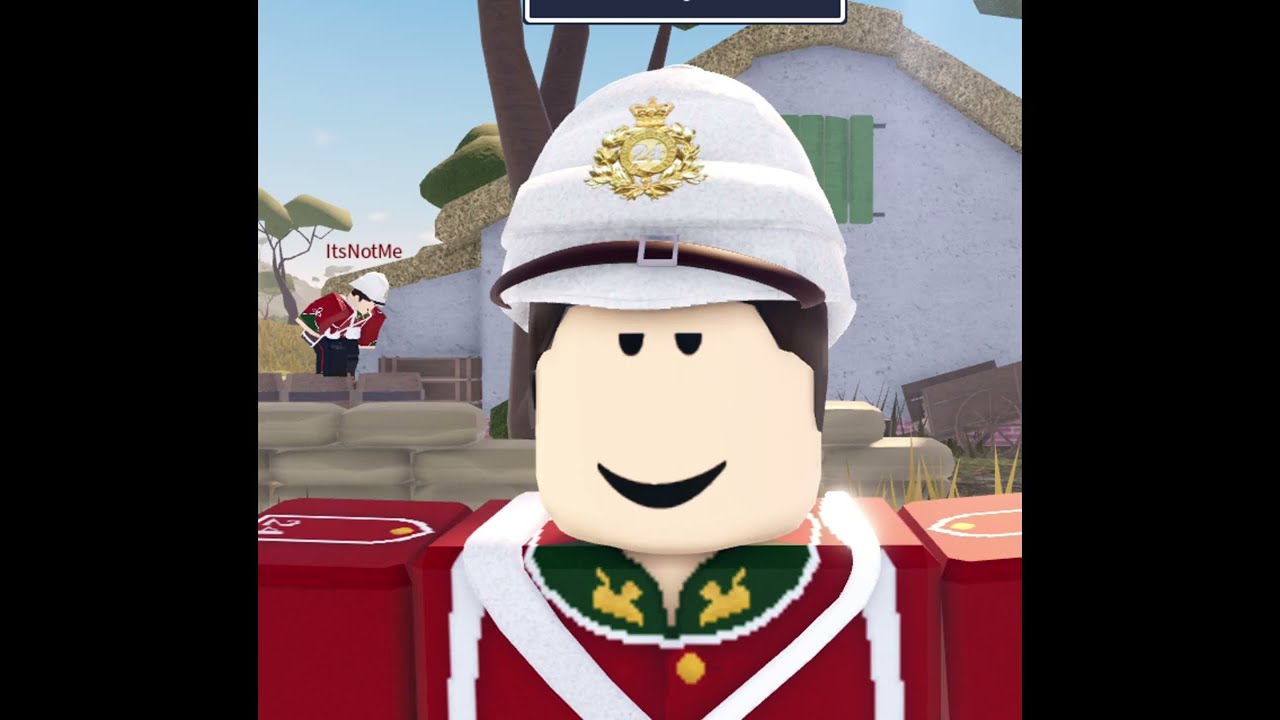The image appears to be a screenshot from an animated video game, resembling characters from Roblox or LEGO. A blocky character occupies the center foreground, notable for his red uniform trimmed with white and gold, and a white hat adorned with a gold emblem. He has dark hair and is smiling. This character exudes a sense of royalty or uniformed authority. Behind him stands another character in a similar getup, looking downwards. Text above this second character’s head reads "It's Not Me." The background displays a picturesque scene featuring a white stucco house with a beige roof, stone or brick walls, and clusters of cartoon trees, set against a clear, sunny blue sky. The overall setting gives the impression of a pastoral or countryside environment.